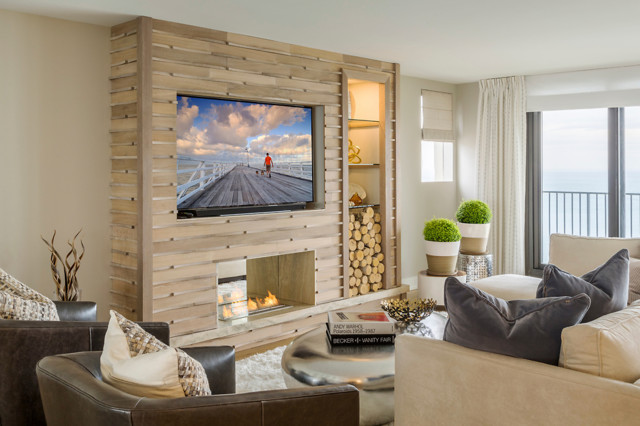This is a detailed, horizontally-oriented photograph capturing the modern and minimalist interior of a coastal home living room during daylight hours. The room features a large set of sliding glass doors on the right, opening up to a railing with a serene view of the ocean and sky, devoid of any trees. The dominant color palette is coastal, with soft, neutral tones providing a calm and inviting atmosphere.

On the left wall of the room is a prominent built-in structure with a driftwood-toned slatted wood design. It houses an electric fireplace at the bottom and an oversized flat-screen TV mounted above it. The TV notably dwarfs the fireplace, and to the right of this setup, there is a vertical built-in unit that serves as a small pantry, complete with logs at the bottom and a few lighted shelves. A small window above this unit features a raised Roman blind, further enhancing the influx of natural light from the open horizontal blinds or drapes on the sliding glass doors.

In the foreground, there are two brown leather armchairs positioned in the lower-left corner, each adorned with large throw pillows. Between them and the fireplace is an oval coffee table, topped with a stack of two books and a bowl. In the lower-right corner sits a white suede sectional sofa with large gray throw pillows, extending toward the sliding glass doors.

Under the small window are two identical round plant stands, each holding a potted plant with tan bottoms and broad white rims, containing rounded green bushes. The overall lighting is bright and natural, emphasizing the cleanliness and modernity of the living space.